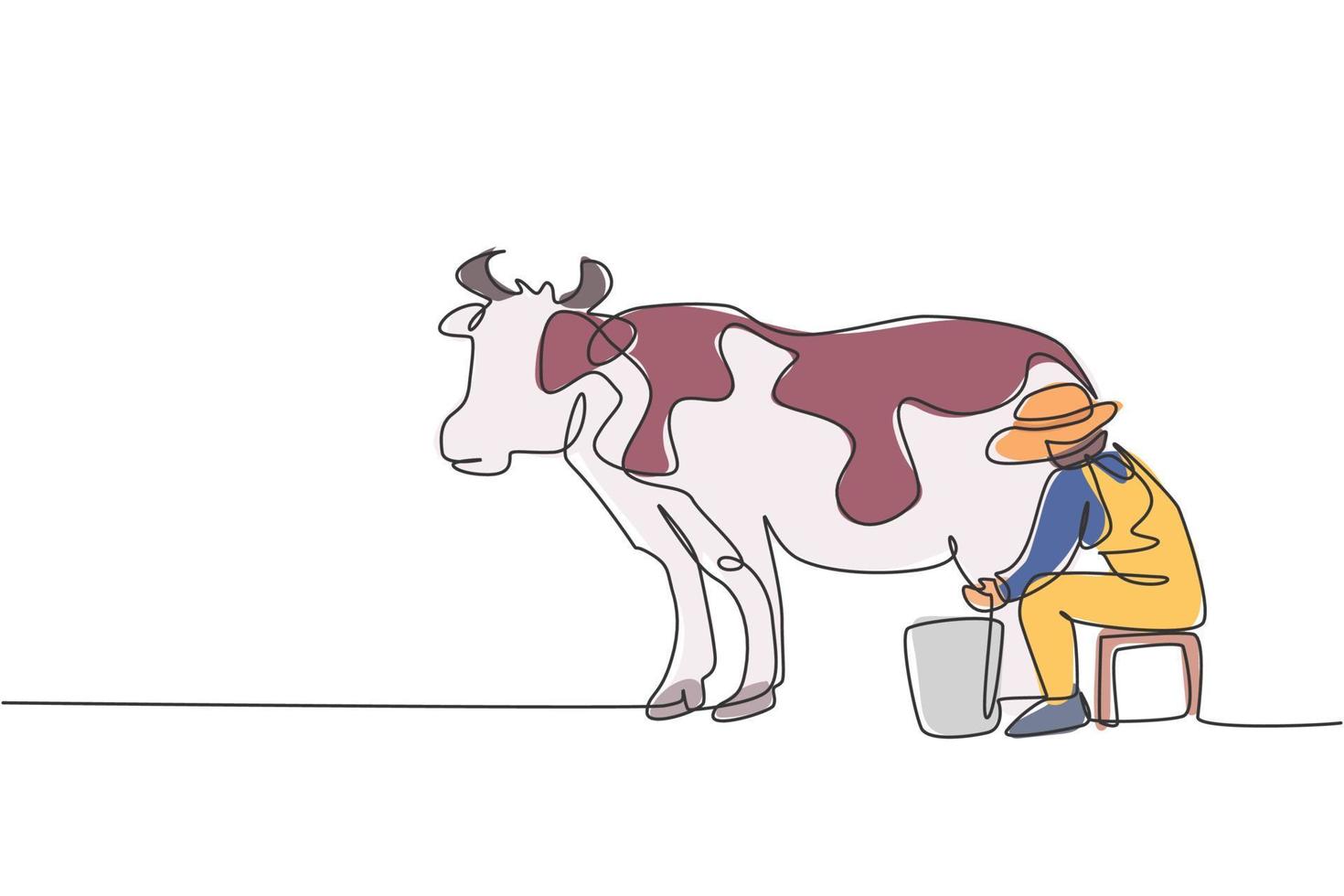The image is an abstract, minimalist cartoon illustration showcasing a man milking a cow. The scene appears to be constructed with a continuous black line that twists and turns to create the entire outline and figures within the image. At the center stands the cow, presented in a unique light pink color with burgundy or reddish-pink spots and two gray horns. The cow lacks facial details like eyes, nose, and mouth, adding to its abstract nature. The man, positioned to the right of the cow, sports yellow overalls over a blue shirt, gray shoes, and a straw or cylindrical-shaped hat. He is seated on a brown stool, concentrating on milking the cow, with his hands placed beneath the udder. A small, gray bucket sits next to him, ready to catch the milk. This blending of continuous line art with the detailed yet simple color palette gives the illustration a distinct, whimsical feel.